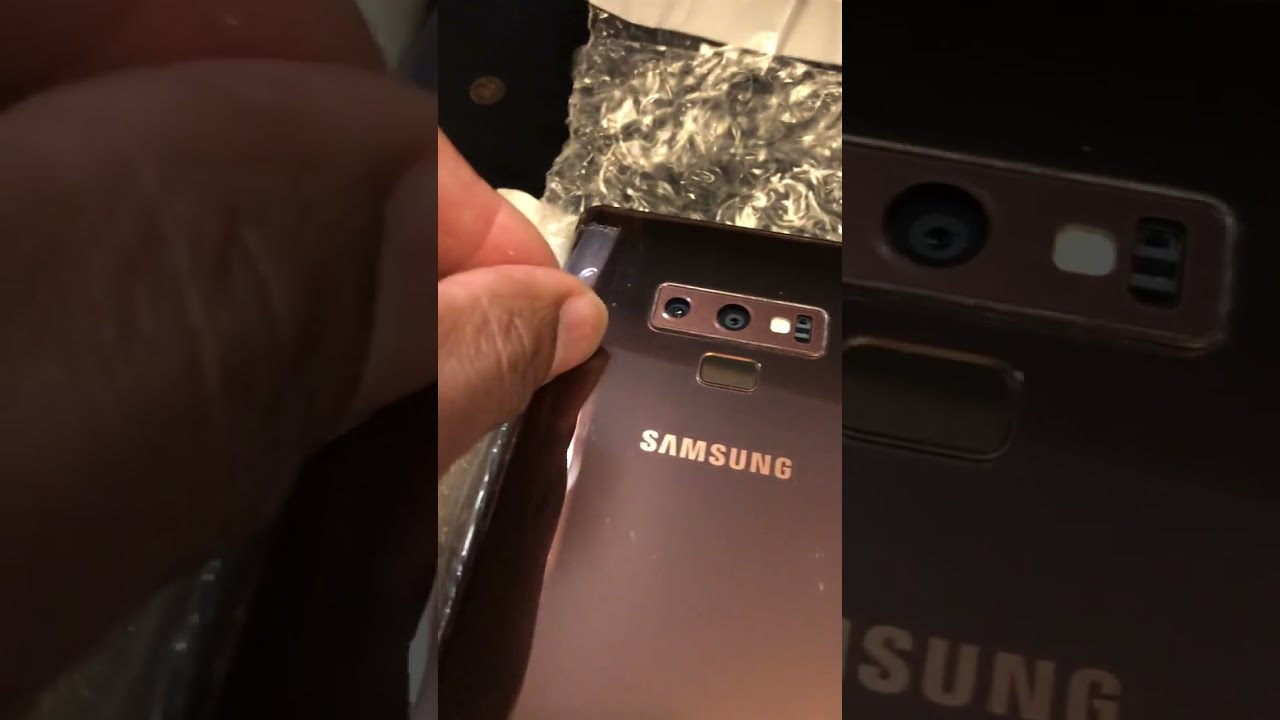The photo features a close-up shot of a Samsung phone with the word "Samsung" clearly visible beneath the centrally located camera. The phone's back shows a configuration of multiple components: a primary camera, a smaller secondary camera on its left, and a white flashlight to its right, with an additional possible third camera further right. Below these elements is a rectangular cutout housing a darker brown button. The image has a black filter, making details hard to discern. In the phone's bottom right corner, there's a white spot likely designed for a phone grip accessory.

The image also shows a person's thumb and index finger on the left, appearing to peel off some packaging tape, suggesting the phone is brand new. This action is further supported by a clear or semi-see-through bag with bubble wrap seen behind the phone. The photograph is divided into three parts: a central photo and magnified border images on the left and right, with the left highlighting the fingers and packaging, and the right featuring a zoomed-in view of the phone and part of the "Samsung" logo. The overall colors in the photo include black, white, brown, and some hints of beige and blue.